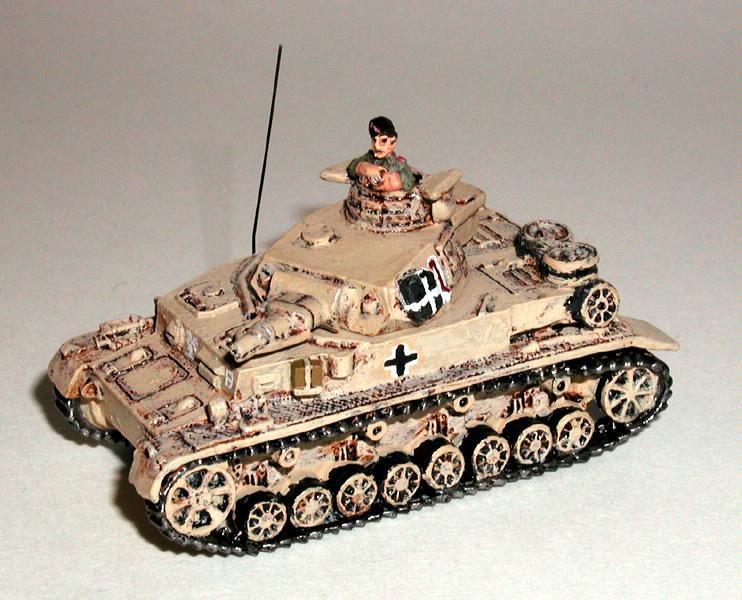The image depicts a meticulously crafted model of a German World War I tank, positioned on a light white or laminate desktop. The tank's body is painted in a beige, desert camouflage pattern, complemented by black metal treads and tan wheels. A striking black antenna protrudes from the vehicle, suggesting it might be a radio-controlled model. Noteworthy features include a black cross, bordered in white, situated prominently on the tank's surface. A soldier figure, adorned in a green shirt and black beret, is seen emerging from the turret, serving as a lookout. The model showcases an impressive attention to detail, with visible gears and components that hint at the tank’s inner mechanics. Despite its high level of craftsmanship, the paintwork appears somewhat uneven, pointing to its likely status as a homemade, do-it-yourself project.